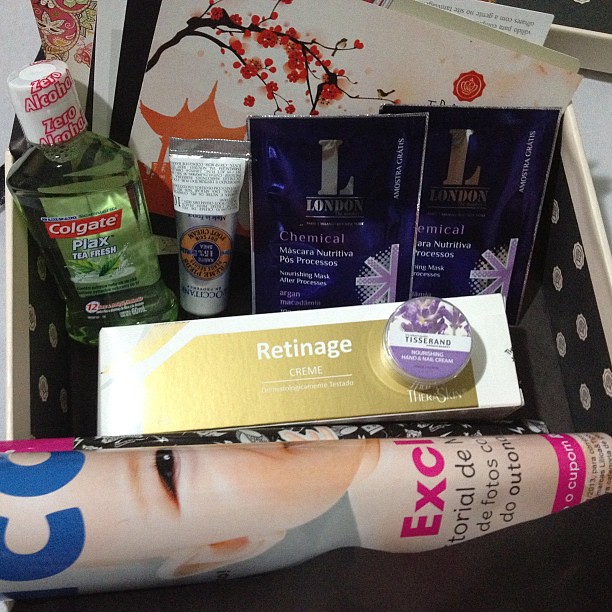The image depicts an open gift box containing an array of beauty and personal care products. The interior of the box is black with white polka dots. Prominently displayed is a clear plastic bottle of Colgate Plax Tea Fresh mouthwash, identifiable by its green liquid. Next to it, there is a silver squeeze tube of L'Occtane hand lotion. The box also contains two purple packages with white text labeled "chemical," alongside a facial mask branded Nutrivita, in a blue package that has "London" written in silver letters at the top.

Additionally, there is a white box adorned with gold shapes, marked with "Retin-Age Cream" in white text. A small round pot with a purple and white design, labeled "Thisserand," is placed atop the Retin-Age Cream box. Included in the ensemble is a partially visible magazine with a cover difficult to read due to its bent position. A few other items featuring designs of cherry blossoms on a tree are also part of this diverse collection.